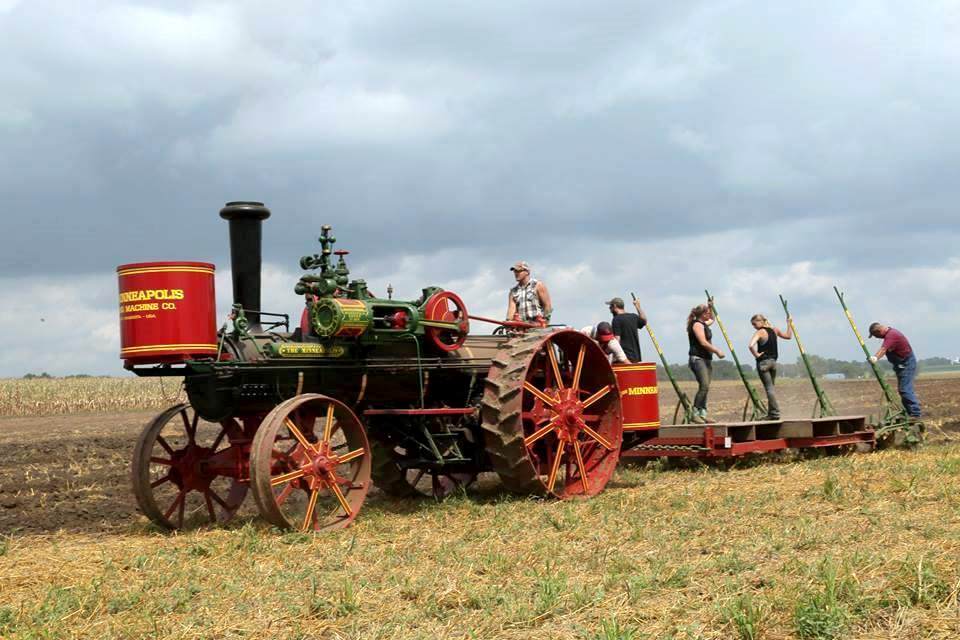The photograph depicts an antique, steam-powered tractor plowing a farmer's field under an ominous, dark sky that threatens rain. The tractor, adorned with massive rear wheels and smaller front wheels both featuring red spoke centers, pulls a low, open-air platform. The platform hosts five workers, their hands occupied with rakes or similar tools, while the driver, a man in a sleeveless flannel shirt and ball cap, steers the tractor. The rear wheels present deep treads and the tractor's engine, characterized by a protruding tall smokestack and gold-accented cylindrical objects, including the word "Minneapolis," hint at its vintage nature. The landscape around them is a mix of plowed earth and patches of green weeds, with some workers handling a red and yellow barrel. The looming, cloud-filled sky adds a dramatic backdrop to this rustic agricultural scene.